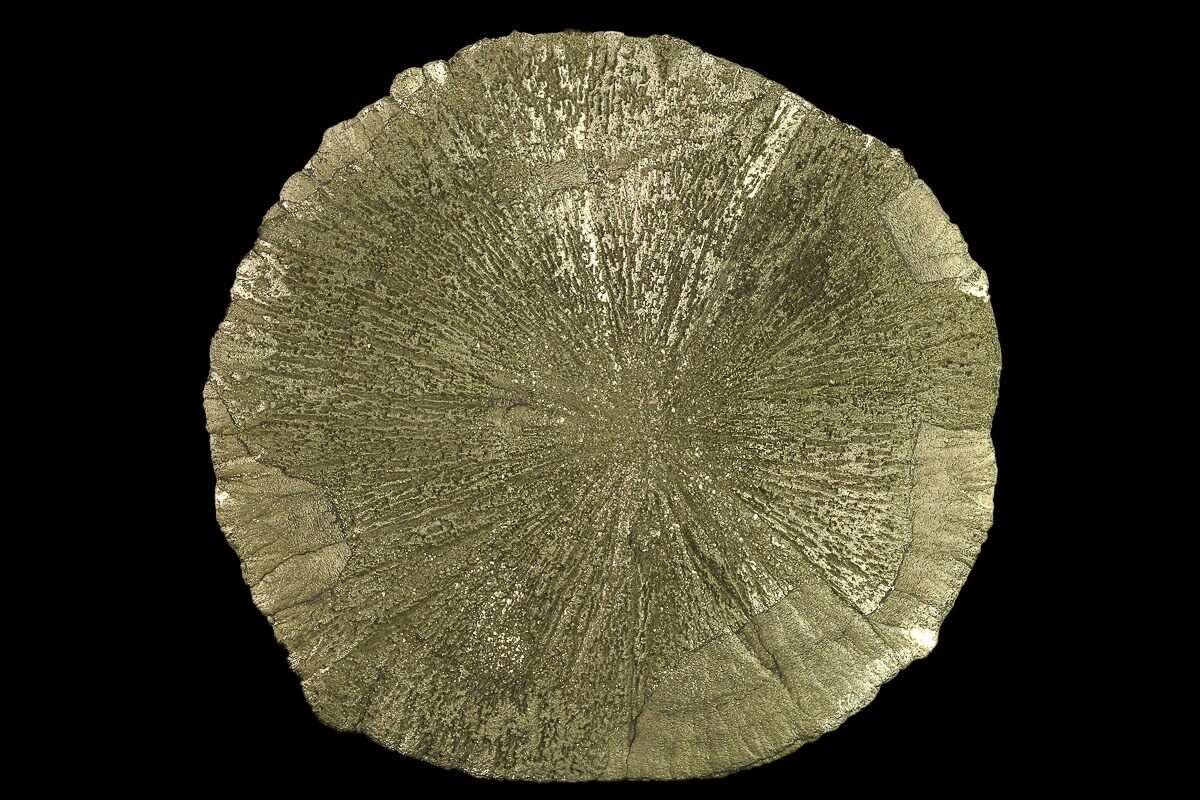This image presents a striking circular object positioned against a large, uniform black background, drawing immediate attention to its intricate details. The object appears to be fossil-like, characterized by a predominantly gray color with various shades of brown, cream, khaki, and ivory. It exhibits a rough, bumpy edge with an elevated, crust-like perimeter. The surface of the object features numerous dark brown lines radiating towards the center, which fade out in some areas to reveal white spots resembling faded rocks. These lines, some of which are dimpled, give the impression of a star-like pattern or the topography of a worn tree trunk viewed from above. Overall, the object’s texture and pattern evoke a sense of ancient, possibly stone-like material, with shell-like impressions, emphasizing its aged and weathered appearance.